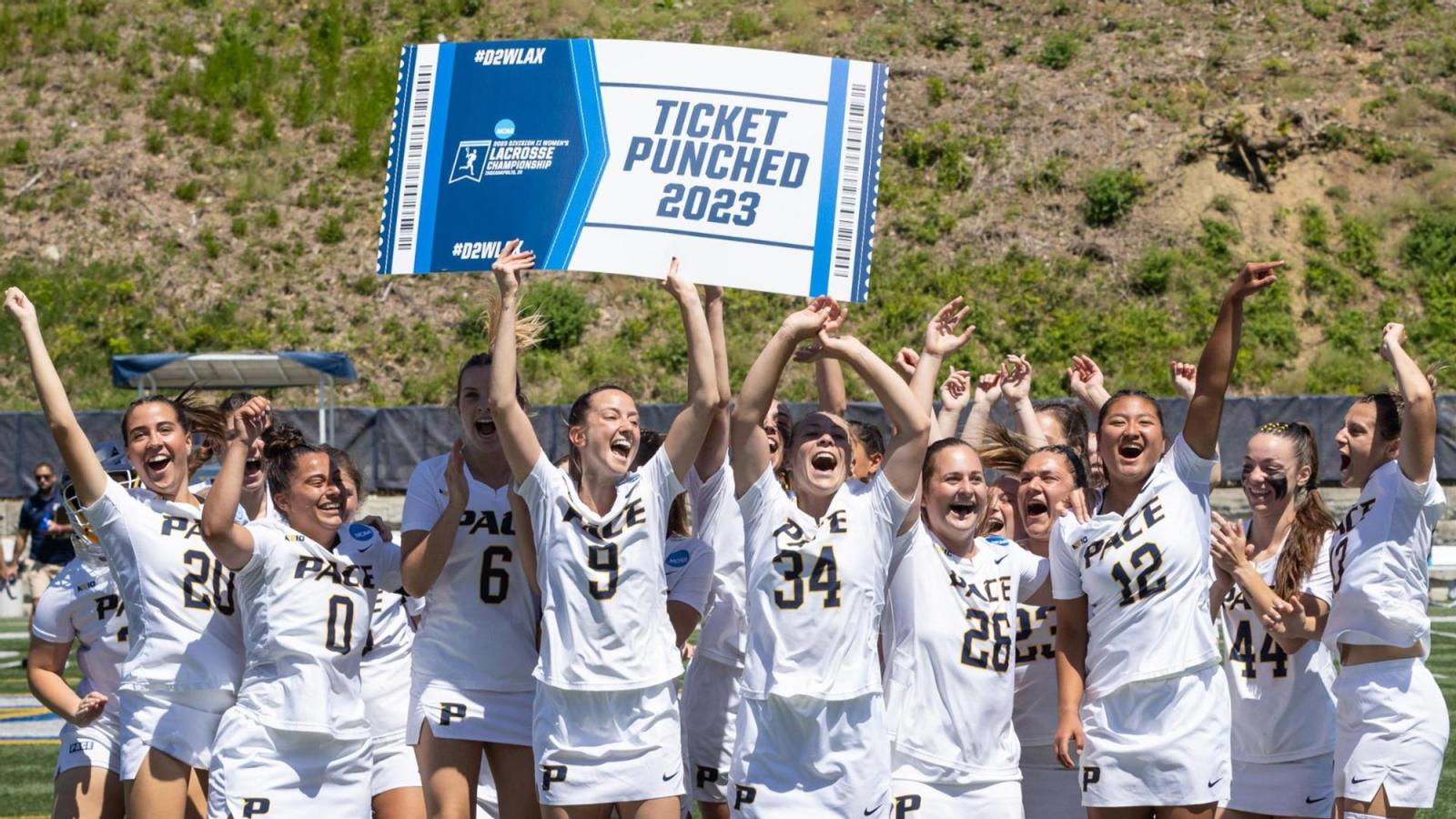The image depicts a jubilant women's lacrosse team, dressed in matching white uniforms emblazoned with "Pace" in dark gray or black font and their individual numbers beneath. The photo, taken outdoors on a sunny day, captures the team celebrating their triumph around a large, blue and white sign designed to resemble a ticket. The sign reads "Ticket Punched 2023" and features the hashtag "#D2WLAX" along with references to the NCAA Women's Lacrosse Championship. The background reveals a dirt and grassy hillside fenced off behind them, indicating the photo was taken near the field where they secured their victory. The players, around twenty in total, are visibly elated, capturing a moment of pure joy and achievement as they hold up their championship ticket.